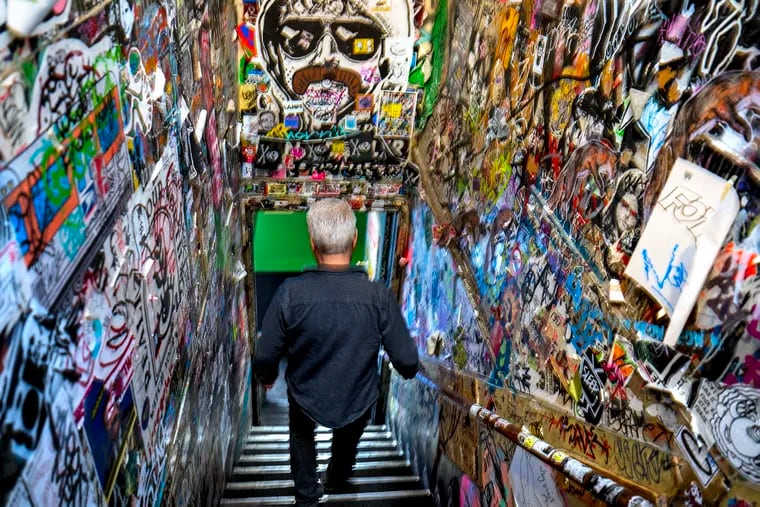In this photograph, an older man with short salt-and-pepper hair is seen from above, descending a staircase. He is dressed in an untucked denim shirt and black pants, gripping the rail adorned with stickers. The stairway is surrounded by walls covered in vibrant and eclectic graffiti and murals. The most notable piece of graffiti is directly above the man's head: a detailed and prominent image of a man in a hoodie wearing aviator sunglasses and sporting a large mustache, evoking a somewhat unsettling, almost iconic presence. The surrounding walls are a kaleidoscope of colors—blue, orange, purple, white, and yellow—contributing to the chaotic, hippie-style aesthetic. Among the graffiti, there are also smaller images, including a depiction of a little girl. The man is walking into or towards a green-colored room, serving as the backdrop to this vivid and intriguing urban art scene.